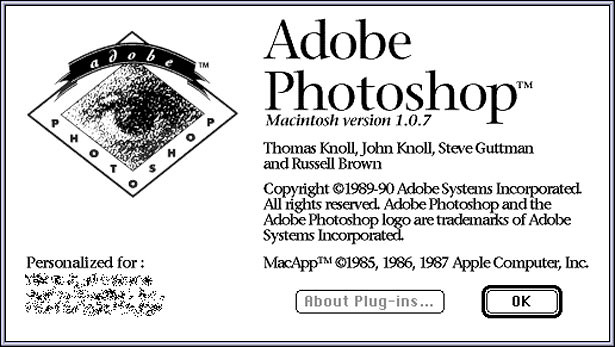The image is a close-up of an old and weathered business card or postcard for Adobe Photoshop, prominently featuring a trademark logo on the left side, which includes a square containing an eye and the text "Adobe Photoshop." The center-right section details the Adobe Photoshop TM Macintosh version 1.0.7, credited to Thomas Knoll, John Knoll, Steve Guttman, and Russell Brown. The card carries a copyright notice from 1989 to 1990 by Adobe Systems Incorporated, with all rights reserved. It mentions Adobe Photoshop and its logo as trademarks of Adobe Systems Incorporated. There's also a reference to an "about plugins" button and an "okay" button, adding a tech interface feel to the vintage document.